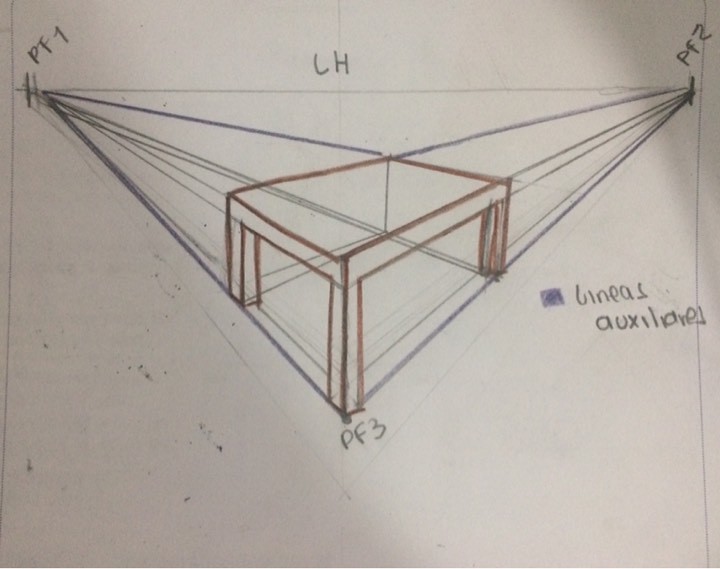The image portrays a detailed architectural sketch, likely a table, drawn on slightly off-white paper using both graphite and colored pencils. The sketch employs a two-point perspective technique, indicative of guidelines extending from vanishing points labeled as PF1 and PF2, denoting "point vanishing" positions on the left and right sides of the drawing. The horizontal line in the background is marked "LH". The table's legs are depicted straight and vertically. Overlaid brown lines highlight the table's wooden rectangular top and legs, making them distinct from the auxiliary guidelines. Notably, there is an inscription of "Lineas Auxiliares", suggesting that the labeling language might be Spanish or French. The sketch shows some erasures and adjustments, indicating refined detailing by the artist. Another marking, PF3, appears, though it does not correspond to a visible third vanishing point, implying a straightforward vertical alignment for the table's legs without convergence.